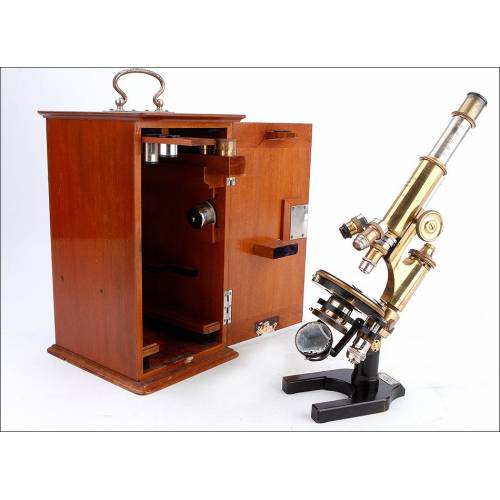The photograph captures a detailed view of an antique microscope set against a stark white background. The microscope, made from a golden-colored metal alloy with silver accents, exudes a vintage charm. It stands on a distinctive horseshoe-shaped black metallic base. The microscope features a flat, round black stage where samples are placed, surrounded by a gray-black circular area for adjustments. Notably, there are three interchangeable lenses protruding from the cylindrical body, highlighting its older design without modern electronic conveniences. 

To the left of the microscope is a sophisticated, reddish-brown wooden cabinet with a shiny finish, likely made from cherry oak. The cabinet door is open, revealing storage space for microscope accessories, and it features a gold-colored handle at the top. The entire setup suggests a piece of scientific equipment from a bygone era, cherished and well-preserved.